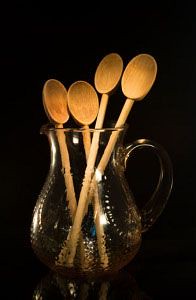This product photography image features a clear glass jug positioned against a fully black background. The jug, shaped like a pot with a curved bottom, a slim top, and a glass handle, is meticulously in focus and brightly lit. Within this glass jug are four wooden spoons, each with a long stem and a smoothly fashioned spoon end. The spoons possess a light brown, tan-like wooden texture. The composition reveals intricate details of the jug, including subtle indentations or decorations, which add to its unique design. The reflective nature of the glass generates a subtle, almost monochromatic interplay with the black background, emphasizing the stark, elegant contrast. The differing lengths of the spoons—two shorter and two longer—break the symmetry, adding an element of casual elegance and practical utility to the scene.